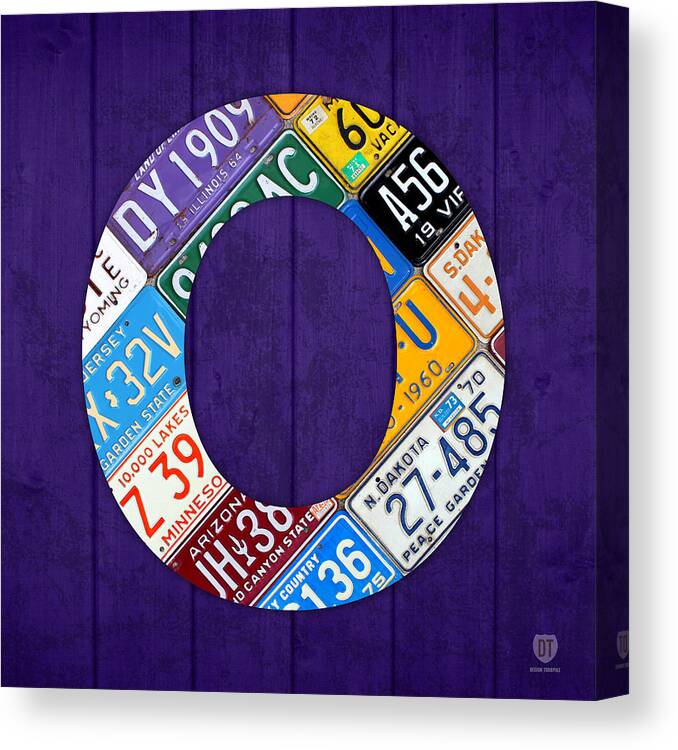The image depicts a canvas wall art hanging against a rich purple fabric background with vertical wood slats and a black border. Centered on the canvas is a large oval "O" made from an eclectic collage of license plates, arranged diagonally from the bottom left to the top right. The vibrant license plates showcase an array of colors including purple, green, blue, orange, red, and white. Several of the visible plates are from various states; one with "Jersey, X, 3, 2, V, Garden State," another from Minnesota with "10,000 Lakes, Z, 3, 9," an Arizona plate displaying "H, 3, 8, Canyon State," a fragment of "North Dakota, 2, 7, 4, 8, 5, Peace Garden," and part of a plate only showing "country, 1, 3, 2." There are also nine other plates with only partial text visible. Additionally, there is a small text reading “DT” in the bottom right corner of the canvas, adding a unique, artistic touch to the piece.